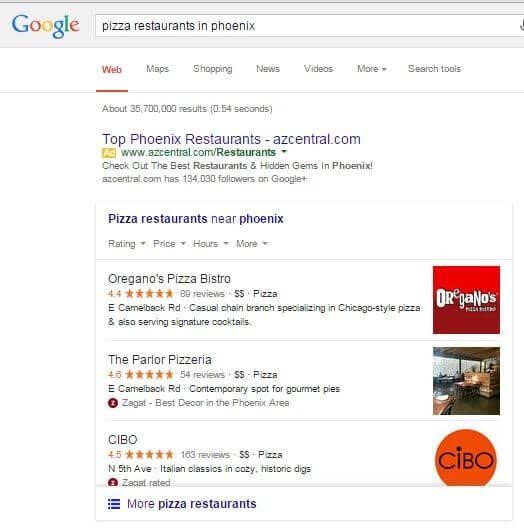A screenshot captures an early 2000s Google search interface displayed on a device. The Google logo in the top left corner is distinctly sharper than the modern, more rounded version, suggesting the interface's age. To the right of the logo is a rectangular search bar characteristic of that era, differing from today's oval shape. Within this search bar, the query "pizza restaurants in Phoenix" appears in a black sans-serif font on a light gray header. A partially visible gray microphone icon is situated towards the right of the search bar.

Beneath the search bar, a series of selectable tabs labeled "Web," "Maps," "Shopping," "News," "Videos," "More" (with a downward arrow), and "Search Tools" are visible. The "Web" tab is distinguished by its bold red font and an underline, while the remaining tabs are in gray. A thin, light gray divider separates these tabs from the search results. Below this divider, in small gray text, is the search result count: "About 35,700,000 results (0.54 seconds)."

The top search result is highlighted in a dark purple, indicating it has previously been clicked. The text reads "Top Phoenix restaurants - azcentral.com." Adjacent to this text, on the left, is a yellow rectangular label with "Ad" in white. Below this is the URL "www.azcentral.com/restaurants," with "restaurants" in bold green and an arrowhead symbol pointing down, hinting at additional menu options.